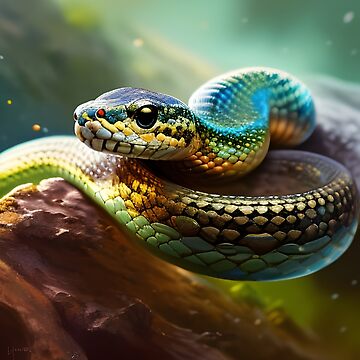This captivating image features a vibrant, computer-generated snake rendered with an intricate and unnatural pattern, resembling a stunning array of gemstones. The snake's shiny, multi-colored scales exhibit sapphire blue, emerald green, gold, rose gold, and pinkish-orange hues. Its underbelly appears to be a bluish-green, while its middle back boasts a striking golden and copper coloration. The snake's head rests slightly elevated on a coil, with its mouth closed and a distinctive red dot on the tip of its nose. Its eyes are black with a reflective blue band at the bottom.

The background of the image is artistically blurred, creating a surreal, almost galactic ambiance with an upper left quadrant of gray and a transition into shades of blue, white, and teal hues towards the upper right. The bottom left features a depiction that could resemble a brown mountain morphing into shades of yellow as it reaches the right corner. The snake appears to be set upon a rock-like formation amidst this vivid backdrop, which also incorporates clouds and a spectrum of colors ranging from yellow to green, to deep blues and oranges. The overall composition gives the impression of the snake majestically resting on a celestial landscape.